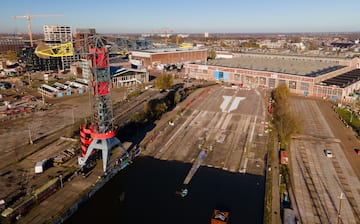The image is an aerial view taken from an altitude of approximately 200 to 300 feet, providing a broad, horizontally oriented perspective of an industrial area on a clear day. The foreground features a vast expanse of brown dirt fields, interspersed with some indistinct vehicles and construction equipment, hinting at an ongoing construction or industrial operation. The lower left foreground is marked by a striking tower-like structure made of grey metal and adorned with red and yellow sections, which appears crane-like but could be part of industrial machinery. There is also mention of railroad cars in this area. 

In the center right, a prominent large building stands, which might be a warehouse or factory, while the background reveals a cityscape with various buildings including some that are potentially residential, as well as taller edifices reaching up to 10 to 15 stories. The distant horizon shows a flat landscape under a blue sky with no mountains, suggesting an expansive suburban or urban sprawl. There is also a canal or waterway hinted at in the dark area near the odd tower. Overall, the image captures a blend of industrial activity and urban infrastructure extending into the distance.